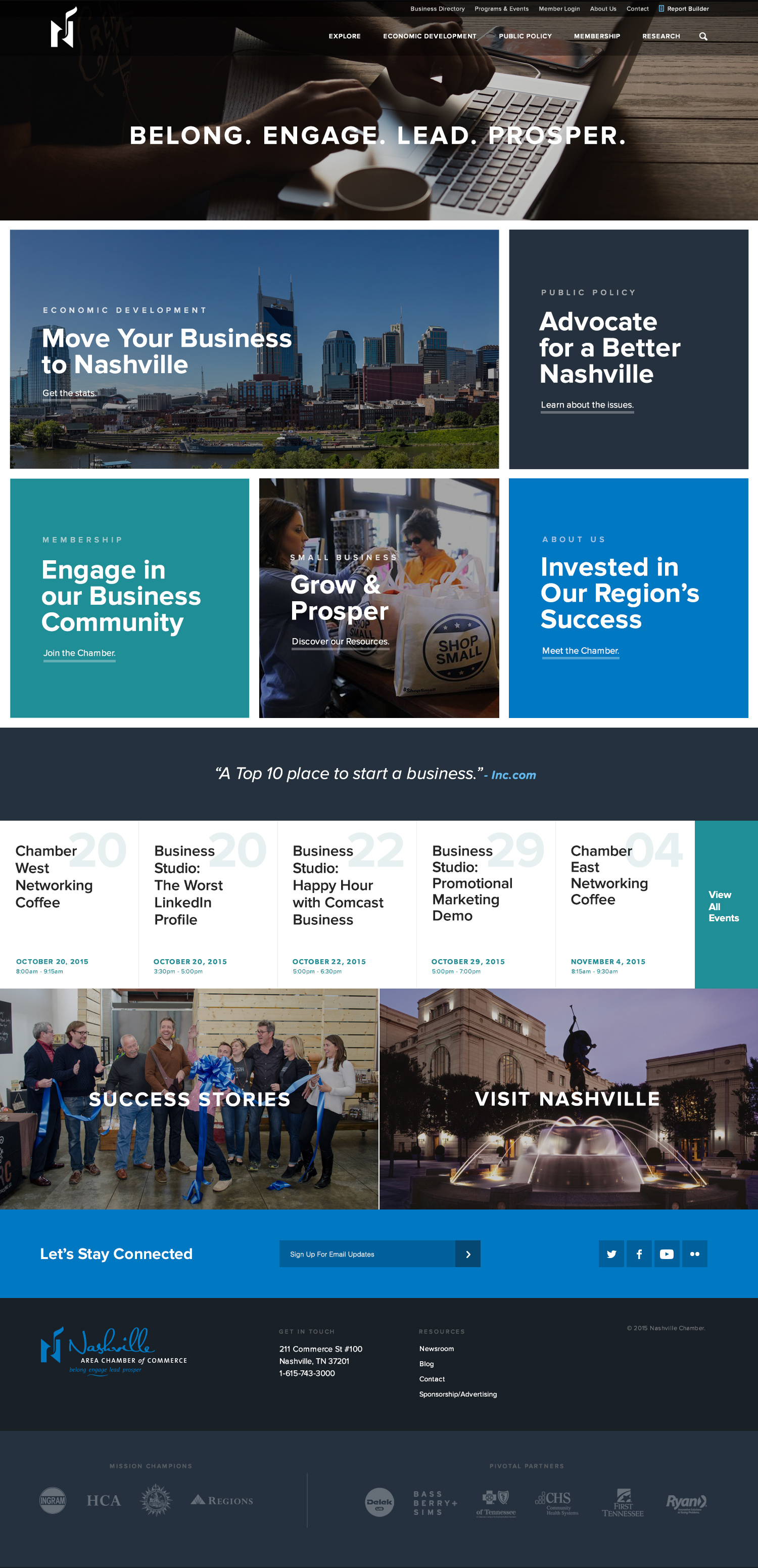A detailed image description for the provided caption could be:

"This image is a screenshot taken from someone's phone, showcasing a webpage filled with various sections promoting business opportunities in Nashville. At the very top, the screen displays encouraging words such as 'belong,' 'engage,' 'lead,' and 'prosper,' layered over a photo of someone typing on a laptop. The person has a cup nearby, ready to start working. Below this, there's a prominent call-to-action box saying: 'Move your business to Nashville, get the stats.' 

Further down, the 'Public Policy' section advocates for a better Nashville, inviting users to 'learn about the issues.' 

Continuing downwards, the 'Membership' section entices individuals to 'engage in our business community' by joining the chamber. Adjacent to this, in the same row, there's a 'Small Business' section encouraging growth and prosperity, depicted with an image of a woman carrying a bag that reads 'shop small.' 

Another section titled 'About Us' highlights the chamber's investment in the region's success. 

Lower down, bold text promotes Nashville as a 'Top 10 Place to Start a Business,' followed by mentions of Chamber West Networking Coffee, Business Studios, 'The Worst LinkedIn Profile,' and a Business Studio happy hour. Finally, there are segments highlighting 'Areas of Success Stories' and an invitation to 'visit Nashville.'"